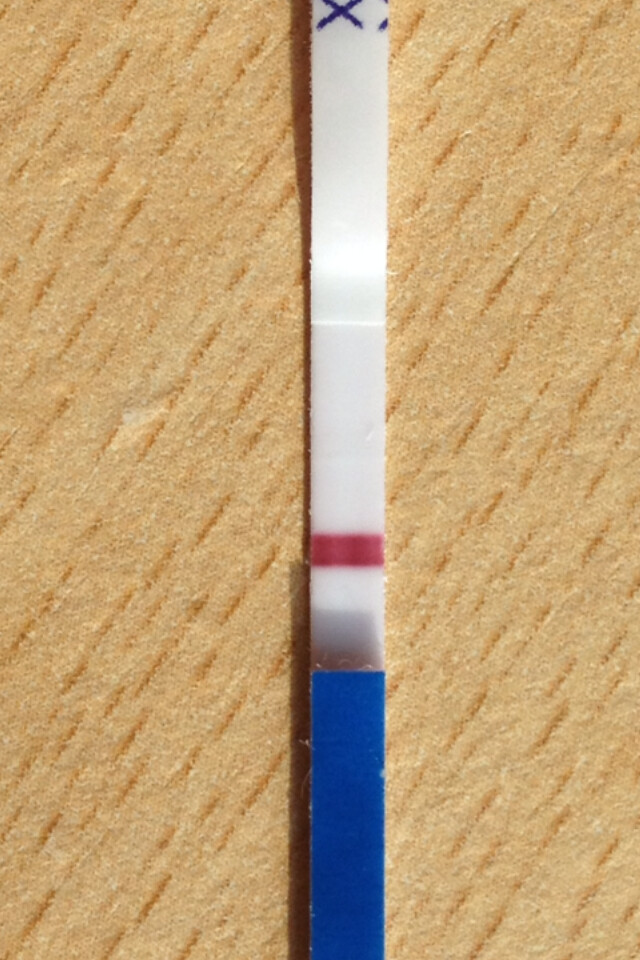The photograph features a central object placed against a background that resembles textured paper with wood chip-like lines, rendered in a dusky pink hue. Prominently positioned in the middle of the image is an object that seems to be either a butter knife, letter opener, or possibly a musical instrument accessory. This object is predominantly white with a red stripe near the handle. The handle itself is a vivid blue, reminiscent of the classic Nokia blue color. A slight shadow is cast from the top of this object, and it is adorned with a black cross at its apex.